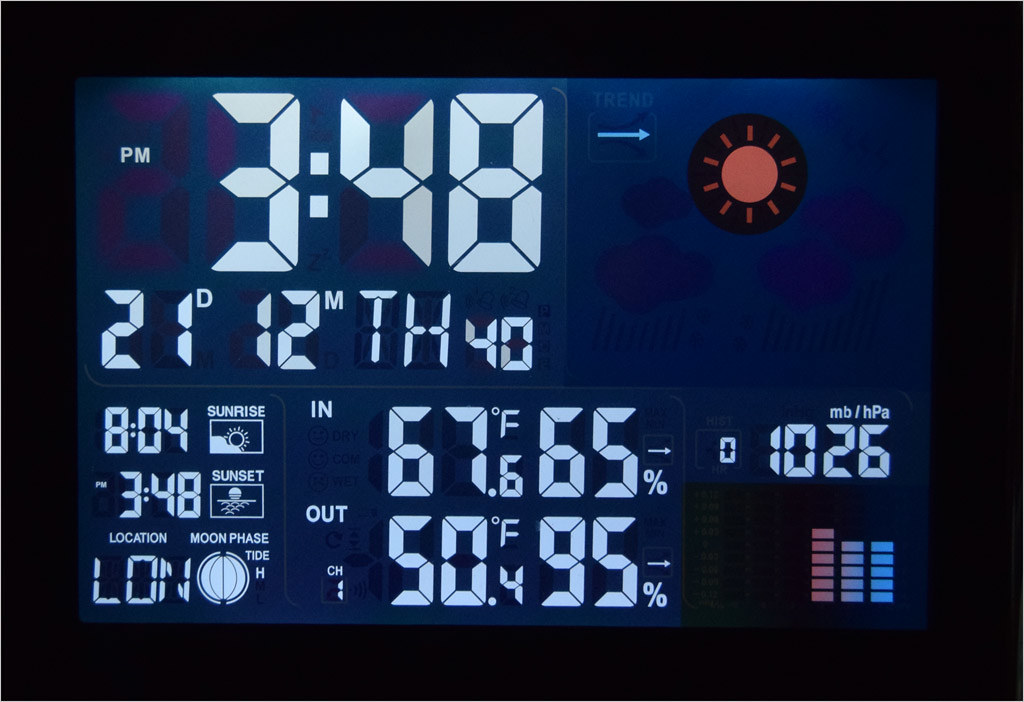A detailed LCD display screenshot from an electronic device showing various weather and time-related readings. The display presents the current time as 3:48 PM on Thursday, December 21st. The weather forecast section includes the time of sunrise at 8:04 AM and sunset at 3:48 PM for the location abbreviated as "LON," likely referring to London. Additionally, it features a diagram illustrating the current moon phase. Temperature readings are given in both indoor and outdoor settings, shown in degrees Fahrenheit, along with the corresponding humidity levels displayed as percentages. The display also includes measurements in millibars (MB) and hectopascals (hPa), enhancing its comprehensive meteorological overview.